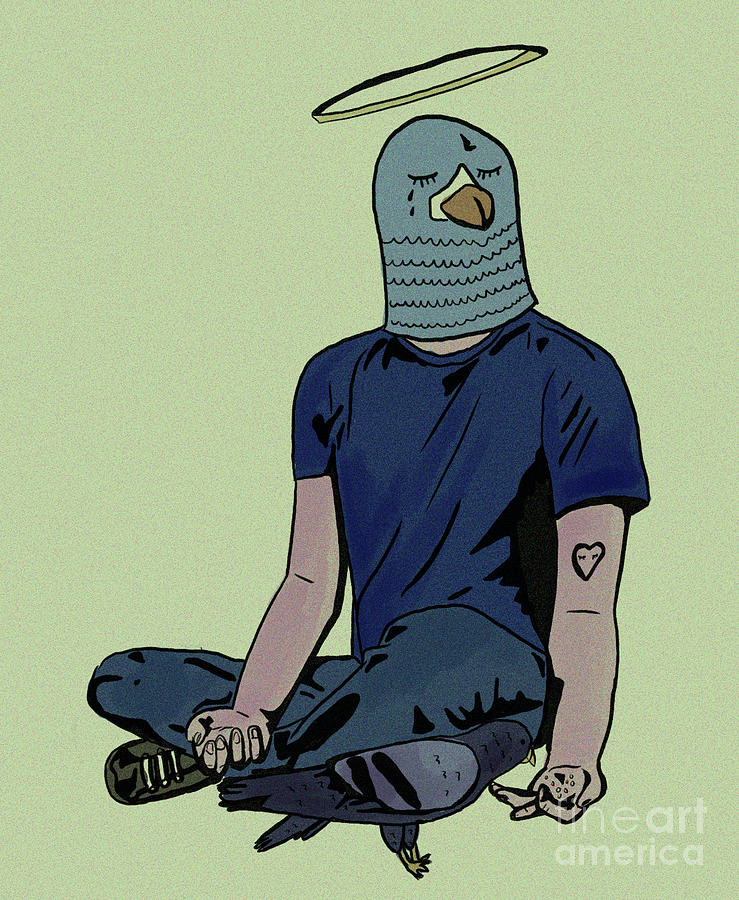The digital painting depicts a young man seated cross-legged against a light sage green background. He is wearing a simple, navy blue short-sleeved shirt, blue jeans, and shoes. On his head is a light green pigeon mask that completely covers his face, and above his head floats a simple black halo. The man’s left arm, which bears a heart-shaped tattoo, is extended outward holding birdseed that a dark blue pigeon is feeding on. His right hand is clenched and resting on his leg. The image is tagged with "Fine Art America" faintly in the bottom left corner. The pigeon mask has closed eyes, with a tear falling from its right eye, adding a layer of poignant symbolism to the scene.